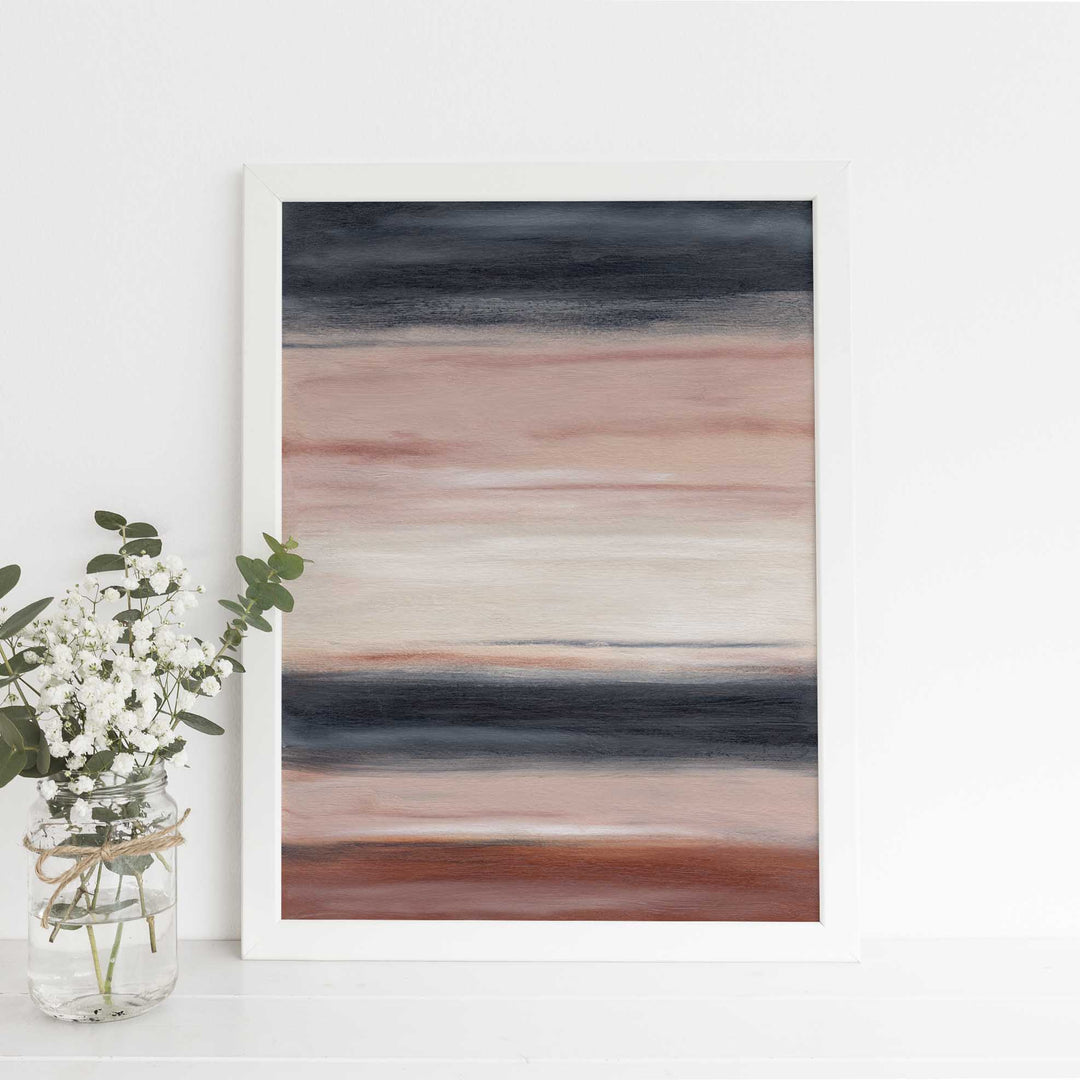This image showcases a painting, tilted against a pristine white wall. The painting is encased in a simple white frame, possibly wooden or plastic. Dominated by thick horizontal layers, the artwork features bands of various colors. From the bottom, the sequence begins with a thick red stripe followed by a whitish-tan layer. Above this, a bold black band intersects the canvas, returning then to another whitish layer with a pinkish hue. The topmost layer reverts to black, forming a pattern of contrasting horizontal lines. The abstract composition may evoke imagery such as sunsets with its array of greens, corals, whites, and dark browns.

Adjacent to this painting, on the same table surface, rests a glass jar. This jar, half-filled with water, sports a decorative bow and contains a live green plant adorned with white flowers, their stems submerged in the water. This carefully selected arrangement complements the serene and abstract nature of the painting, creating a cohesive and visually pleasing scene.